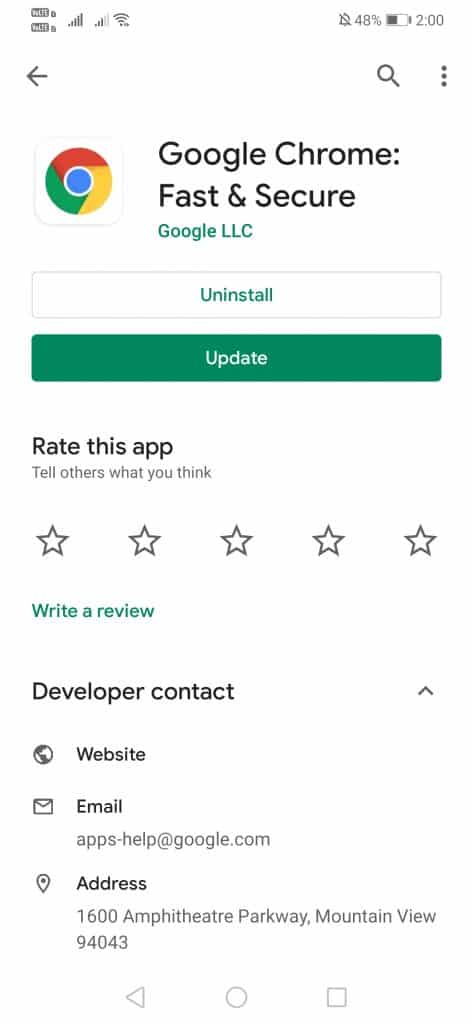This image is a detailed screenshot of a smartphone displaying a web page from the Google Play Store. The screen features a white background with the smartphone's standard top bar showing the battery life, current time, and internet connection status. Directly beneath this is a navigation bar for web browsing. Prominently displayed just below the navigation bar, the text "Google Chrome: Fast & Secure" appears in bold black letters, accompanied by the recognizable Google icon on its left. 

Two prominent buttons labeled "Uninstall" and "Update" are situated directly underneath, indicating that the user is viewing the app page for Google Chrome. This is further confirmed by the presence of the "Rate This App" section below these buttons, which allows users to rate the app by selecting from one to five stars. Further down, the page provides additional information where users can find help and contact Google support for assistance. The overall layout and content strongly suggest that this is a screenshot of the Google Chrome app page within the Google Play Store.